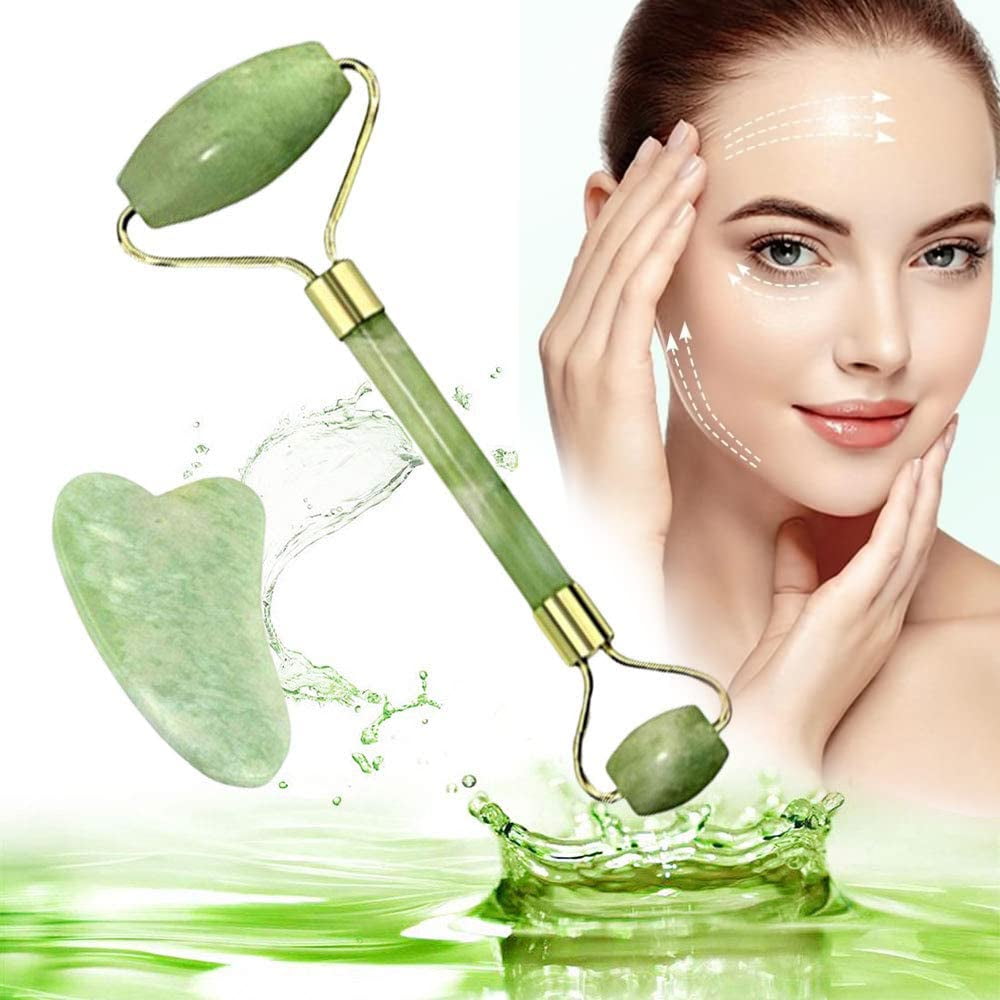In this vibrant skincare advertisement, a young woman with fair, smooth skin, and brownish-red hair styled in an updo gazes confidently from the upper right corner. Her striking presence is accentuated by pink lipstick and expressive eyes. Her left hand gently supports her jawline while her right hand cups her cheek, illustrating a thoughtful and poised demeanor. Arrows annotate her forehead, under-eye areas, and chin, highlighting the targeted skincare routine. To the left of her, a green emerald-like face stick and a green gua sha tool are displayed, emerging from a pool of green-tinted water with splashes accentuating their freshness and vitality. The face stick features a translucent green cylindrical handle with prominent roller beads at each end, designed for facial massage and skincare application. This scene is set against a pristine white background, enhancing the vibrant green of the products and the serene yet invigorating atmosphere of the image.